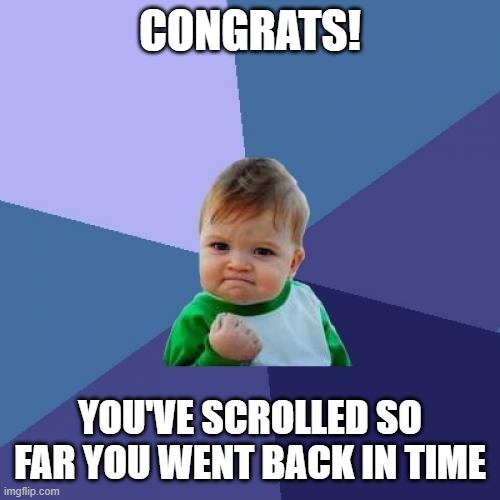The meme features a square background with an ornate, circular pattern made up of numerous triangular sections. These sections showcase varying shades of purple and blue, which create a visually vibrant and engaging design that resembles slices of pizza. 

At the center of this intricate background, a toddler's face is prominently displayed. The child has light brown, almost blond hair, and dark eyes. The expression on the toddler's face is one of determination, with their mouth and jaw clenched tightly and a small fist raised close to their face. The toddler, who appears to be Caucasian, is wearing a green-collared t-shirt with green sleeves and a white chest.

Overlaying this image, there is bold text with a black outline. At the top of the meme, it reads "CONGRATS!" in white, capital letters, followed by an exclamation point. Below the toddler's face, additional text in all capital letters states, "YOU'VE SCROLLED SO FAR, YOU WENT BACK IN TIME." The toddler's determined expression, coupled with the strong, motivational text, adds a humorous and engaging touch to the vibrant, multi-colored backdrop.